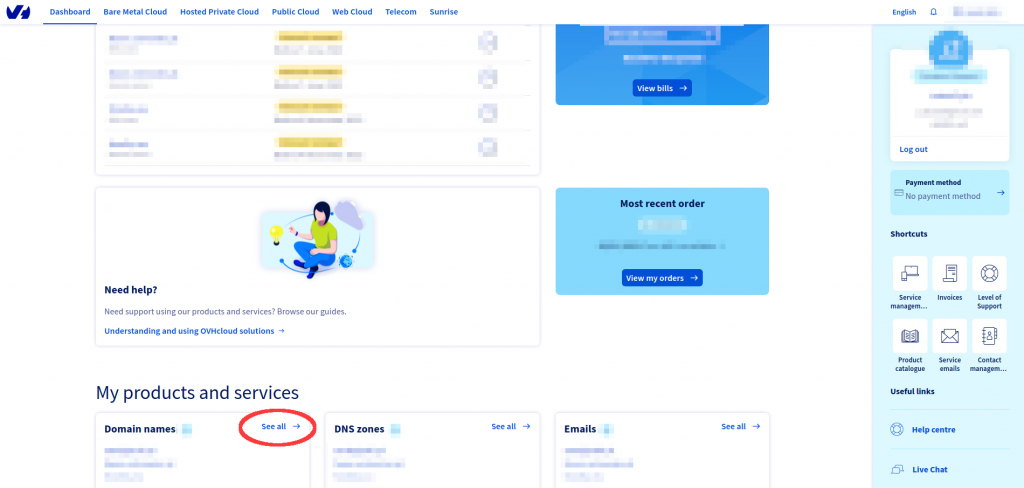In the image, we observe a comprehensive dashboard teeming with various cloud computing services and functionalities. Dominating the top section is a list that includes categories such as "Bare Metal Cloud," "Private Cloud," "Public Cloud," "Web Cloud," and "Telecom." The entire scene is intentionally blurred, contributing to a subtle, mystifying ambiance, especially noticeable during the sunrise backdrop.

Blue bars prominently labeled "View Bills" and "My Orders" are positioned towards the center and right side of the frame, directing attention to the financial and transactional aspects of the dashboard. The center displays a slightly pixelated figure sitting, while the adjacent right sections indicate the most recent orders, also characterized by a high degree of pixelation.

Around the dashboard, we find various sections aiming to provide assistance and guides: "Need Help," "Need Support Using Private Services," and "Browser Guides" along with "Understanding OVH Cloud Solutions." These are complemented by detailed listings of "My Products and Services," which seem to include domain-related elements like "Domain Names, CL," "DNS Zones, CL," and "Emails, Success CL."

Further to the right, an even more pixelated segment appears, indicating payment methods. The text notes the absence of a payment method setup. Additional tools and navigation aids scattered across the interface include "Shortcuts," "Service Management," "Invoices," "Level of Support," "Product," "Service," "Emails," "Useful Links," "Help Center," and "Live Chat."

The dashboard, though blurry and pixelated, is meticulously categorized, providing a rich canvas of the user's cloud management ecosystem.